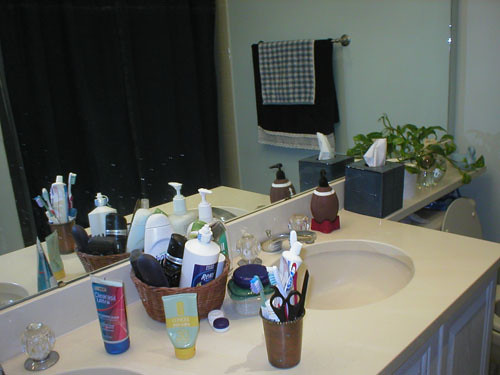This photograph captures a corner of a bathroom with various details. At its center is a brown double sink unit, prominently displayed in the middle and lower left of the image. The sink, adorned with gold-colored fixtures and glass-like plastic knobs for hot and cold water, is cluttered with several items: upside-down bottles, a basket filled with more bottles, and a cup containing scissors, toothpaste, and toothbrushes. A small football-shaped lotion dispenser is positioned on its end, with a nozzle at the top.

In the background, part of a toilet is visible, featuring a box of Kleenex and a plant in a glass dish placed above the tank. The green wall holds a fixture from which two towels hang, one dark and one lighter, their reflections caught in the large mirror above the sink. White cabinets, located below the sink unit, provide a sharp contrast to the overall brown and gold theme of the sink area. The photograph offers a detailed glimpse into the functional and decorative elements of this bathroom space.